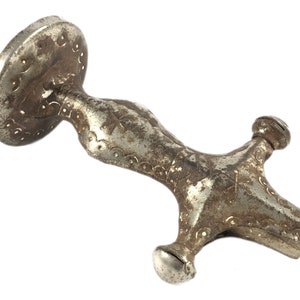This image depicts the ornate handle and partial base of a sword against a white background. The handle, primarily metallic in appearance, appears aged with a mix of silver and tarnished, possibly gold, details. Starting at the base, which has a flat circular section where the blade would extend, the handle features intricate designs including squiggly lines, circles, and dots. This decorative pattern continues up the handle, which bulges and narrows with a bulbous area for gripping. At the top, two protrusions jut out to form a crossguard. The entirety of the visible sword is adorned with these elaborate etchings and ornamentation. The intricate patterns and tarnish suggest it is an antique piece, with its true splendor somewhat obscured by age. The photo cuts off the remaining length of the blade, offering only a glimpse into this beautifully crafted item.